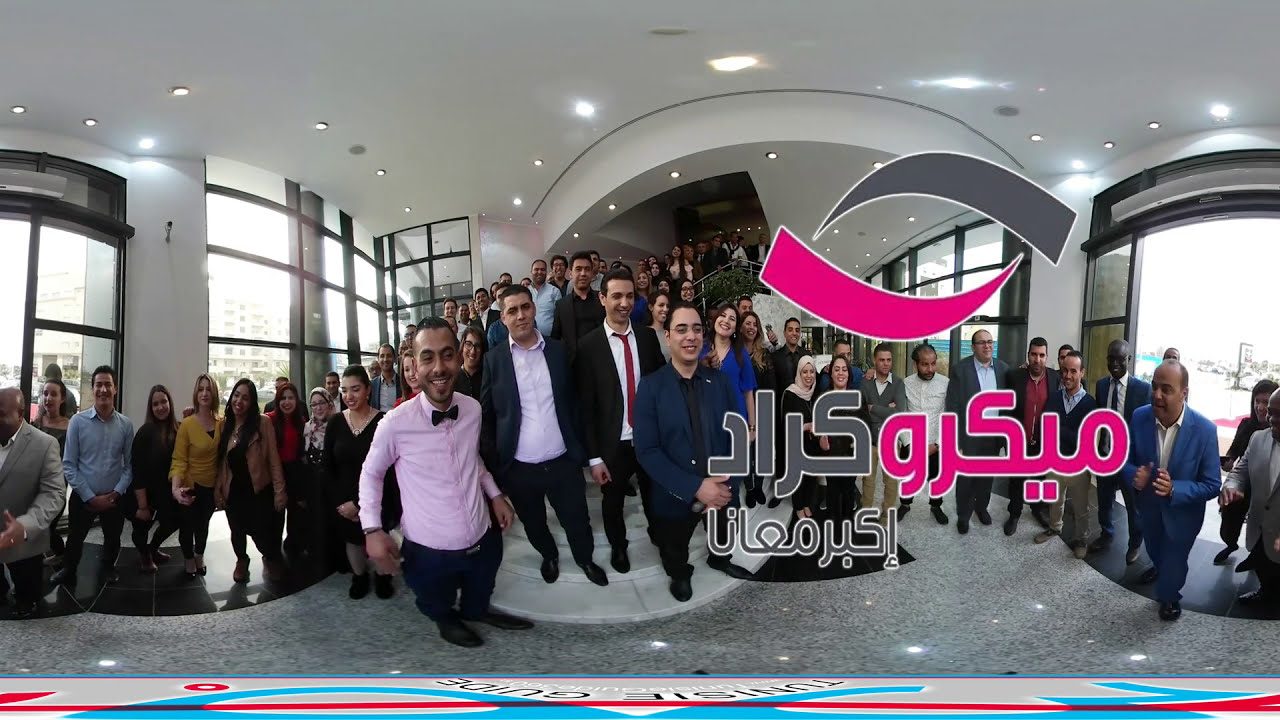The image depicts a large corporate gathering in a modern, upscale office building with a tall ceiling and numerous windows allowing an abundance of natural light to flood in. The venue appears to have multiple floors, with a wide staircase leading to the second level, which is also populated by individuals. The photo features well over 100 people, all dressed in business casual or formal attire, including suits, ties, and headscarves. There is a festive, joyous atmosphere as most individuals are smiling and posing for the picture. The setting is furnished with grey flooring, enhancing the modern aesthetic. Overlaying the image is a logo with a pink and grey swoosh, accompanied by text in a non-Roman script, possibly Arabic or another Middle Eastern or Asian language, indicating the company’s identity.